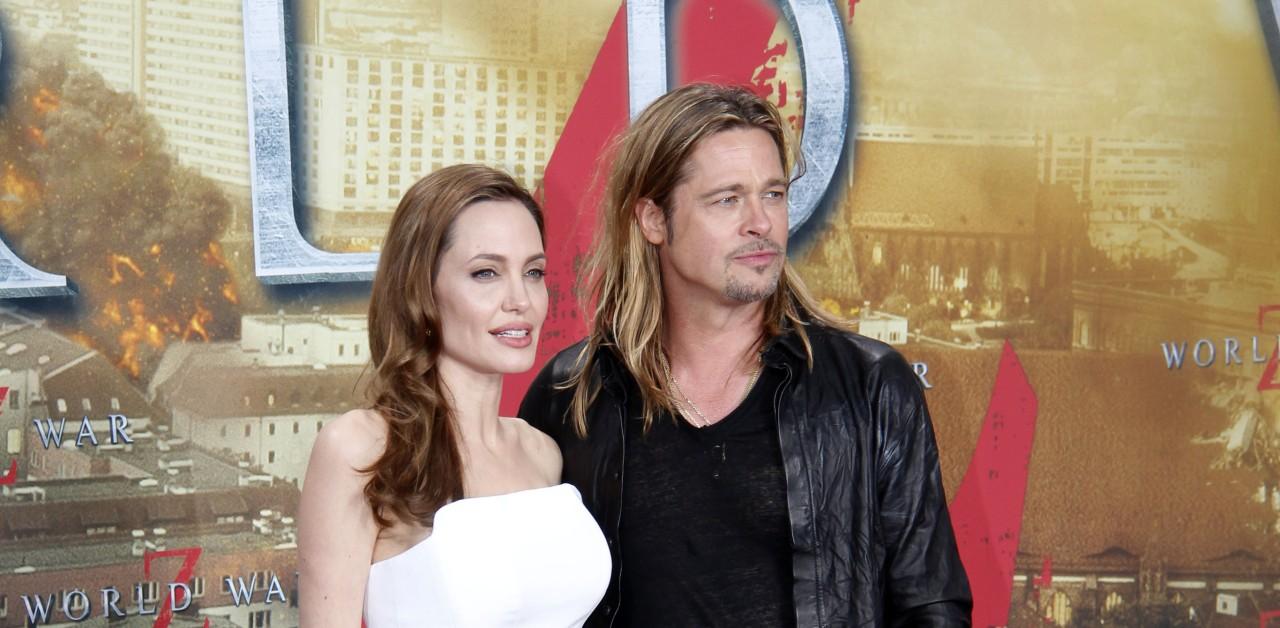In the photograph, Brad Pitt and Angelina Jolie are posing at what appears to be a red carpet event, notably in front of a backdrop for "World War Z." The background features a dramatic scene with buildings engulfed in fire and smoke, large red Z's, and the title "World War Z" prominently displayed in white block font. Angelina stands on the left with her light brown hair draped over her right shoulder. She is dressed in a strapless white evening gown. To her right stands a younger Brad Pitt sporting long, blonde hair. He is dressed in a black V-neck t-shirt layered with a black leather jacket. Although the image captures them from the chest up, the vivid backdrop and their elegant attire create a striking composition.